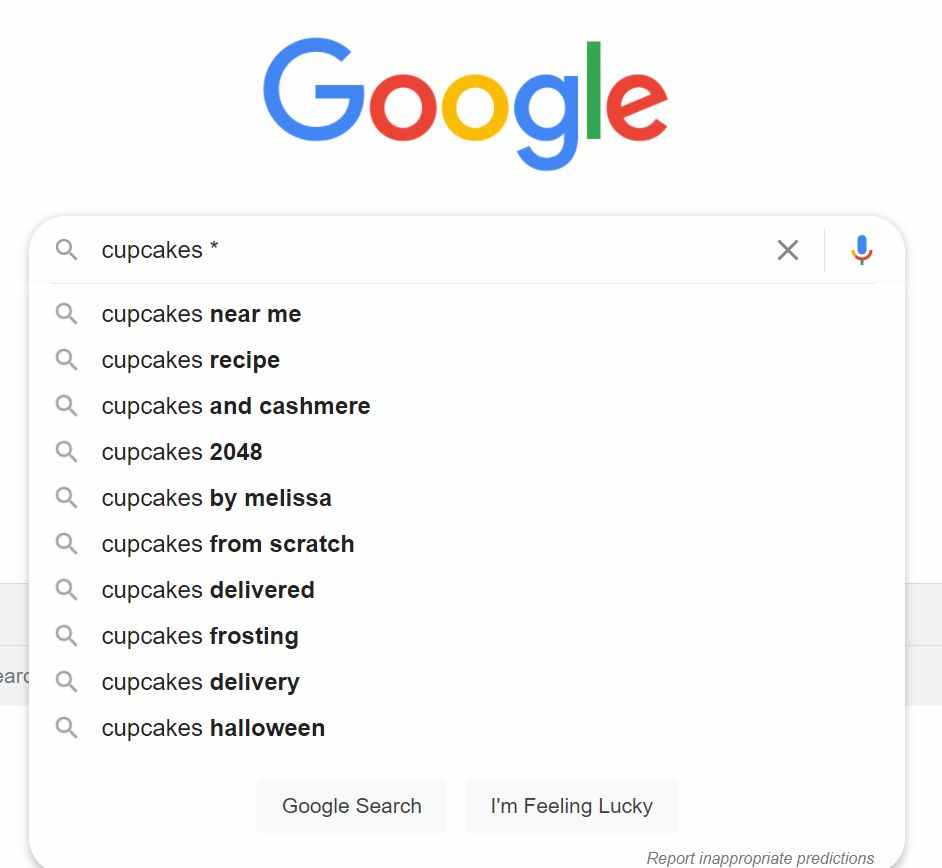The image is a screenshot of a Google search page. At the top, the iconic Google logo is displayed, featuring a blue uppercase "G," a red lowercase "o," a yellow lowercase "o," a blue lowercase "g," a green lowercase "l," and a red lowercase "e." Beneath the logo is the search bar, within which the word "cupcakes" is typed, followed by an asterisk. The search bar contains a blue-colored microphone icon on the right side, indicative of the voice search option, and an "X" icon within the text box for clearing the text.

Below the search bar, a list of suggested search terms is presented, all written in black text on a white background. The suggestions include:

- cupcakes near me
- cupcakes recipe
- cupcakes and cashmere
- cupcakes 2048
- cupcakes by Melissa
- cupcakes from scratch
- cupcakes delivered
- cupcakes frosting
- cupcakes delivery
- cupcakes Halloween

Under these suggestions, there are two rectangular buttons. The left button says "Google Search," while the right one, which is gray with black text, says "I'm Feeling Lucky." At the bottom, in small gray text, the option to "Report inappropriate predictions" is visible.